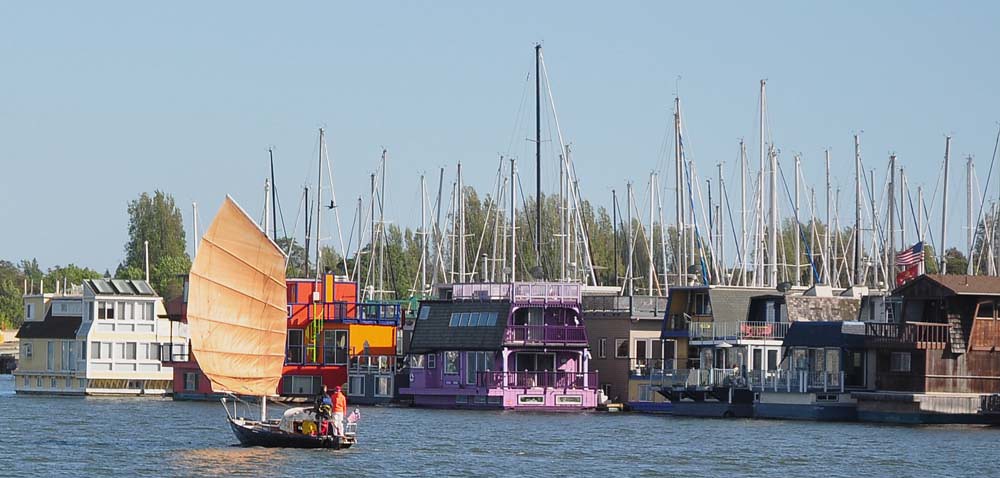The image is a vibrant, outdoor, landscape-oriented photograph taken on a clear blue sunny day, without a cloud in the sky. The scene depicts a tranquil waterway with strikingly blue water. In the foreground, a sailboat with a large, tan rectangular sail floats on the water, manned by two blurry figures—one dressed in orange, the other in blue. 

Docked behind the sailboat is a colorful array of six houseboats, each unique in coloration and design. The first houseboat on the right is brown and wooden, adorned with both an American flag and a smaller red flag beneath it. The next is white with a blue roof, followed by a gray houseboat with a brown roof. A purple houseboat with a gray roof follows, succeeded by an orange and yellow houseboat featuring a green and purple fence. The last in the row is tan with a brown roof. 

Each houseboat is equipped with tall, metal power pole-like structures extending skyward. The background is framed by a peaceful vista of distant trees, adding to the serene, picturesque quality of the scene.